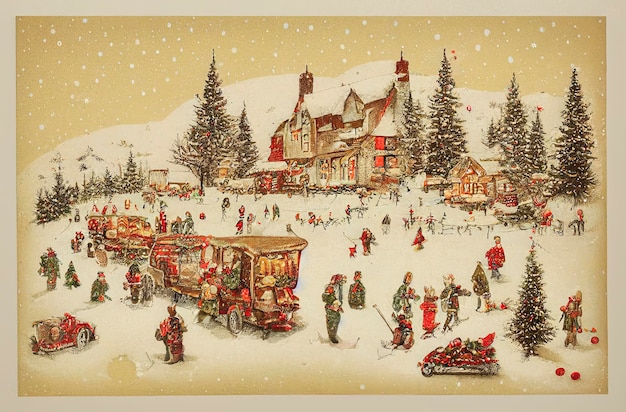This captivating winter scene, reminiscent of a greeting card, depicts a festive and bustling Christmas setting. In the center, a large house or cottage is nestled halfway up a snow-covered hill, surrounded by tall pine trees dusted with snow. Above the cottage, mountain peaks rise into a sky filled with delicate white snowflakes falling gently against a beige or tan background.

The scene is alive with activity. Families and children, all clad in green and red attire, are joyfully playing in the snow and engaging in sleigh rides. In the foreground, a small market offers Christmas goods, adding to the festive atmosphere. Various vehicles, including buggies and sleighs, decorated with wreaths and red bows, are scattered around the snowy landscape. People are seen chatting and mingling near the vehicles and around the larger building, enhancing the sense of community and holiday cheer.